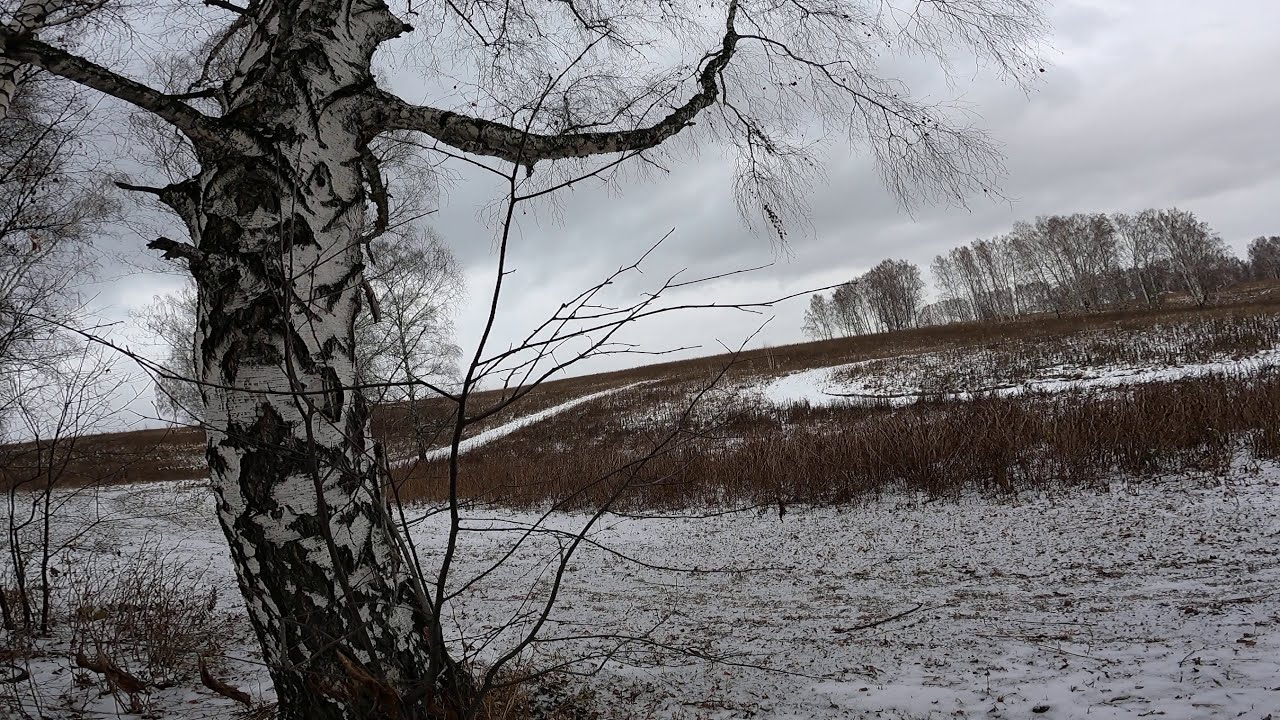This outdoor color photograph in landscape orientation captures a serene and wintry scene at the bottom of a snow-blanketed hill. A dirt road, now covered in snow, begins at the lower right-hand side of the image, cuts across to the left, and makes a sharp turn upwards, weaving into the hillside. To the left of this snowy path stands a large birch tree with a distinctive leaning trunk, covered in a mixture of thick black and white bark. The tree, devoid of leaves, features two prominent branches reaching out in opposite directions near the top, with delicate, sparse branches adorning the lower half.

The barren hillside is peppered with scattered, deep brown weeds and grasses, adding contrast to the whiteness of the snow. Atop the hill, a row of stark, leafless trees stands against a gray, cloud-filled sky, characteristic of a typical winter's day. In the foreground, another snow-covered trail forms a circular shape on the hillside, encircling a cluster of dead trees. The overall scene is a vivid and detailed representation of winter's quiet beauty, encapsulating the stillness and stark contrasts of a snowy day.